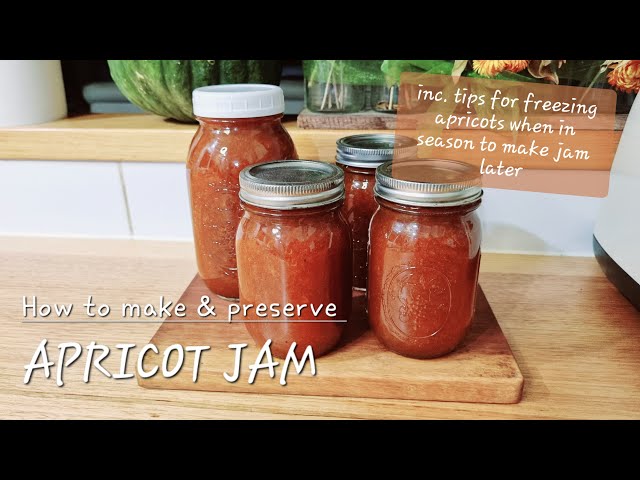This vibrant color photo prominently features four glass jars filled with a rich, dark red apricot jam. Positioned symmetrically in a two-by-two arrangement, three of the jars are capped with twisty silver metal lids, while the tallest jar in the back row features a distinct white plastic cover. These jars are displayed on a small, square-shaped wooden cutting board, itself resting on a larger wooden counter.

In the bottom left corner of the photograph, white lettering reads "How to Make and Preserve," with an additional line below in larger font stating "apricot jam." In the upper right corner, white text on an orange-translucent sign further provides "INC. tips for freezing apricots when in season to make jam later."

The backdrop reveals a cozy kitchen scene: a large, ridged green vegetable that resembles a watermelon or pumpkin sits on a shelf, flanked by jars containing various items. Among these are white stalks and greenery in one jar, and a couple of pinkish-yellow flowers, possibly wilting, adding a touch of organic beauty to the composition. Above, a wooden shelf holds more kitchen essentials and appliances, contributing to the rustic ambiance of the setting.